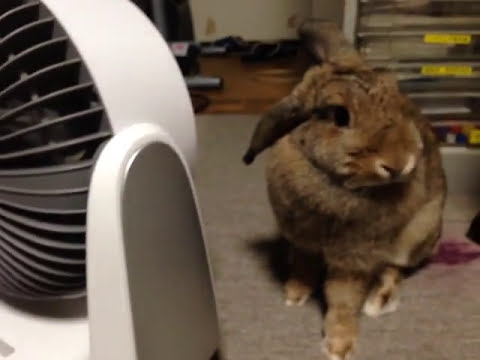In this picture, a predominantly brown bunny rabbit with spots of white and gray fur sits on a gray mat or brownish-gray table, looking slightly to the left, giving us a frontal view. Its left ear hangs down while the right ear sticks straight back. The background features a wooden floor and some indistinct objects, possibly including metal shelving. Directly to the left of the bunny, a small white portable electric fan with gray venting and black grates blows air towards the rabbit. The image is indoors, devoid of any people or text, and includes other varied shades and small objects whose details are hard to discern. The scene centers on the rabbit, comfortably sitting in front of the fan.